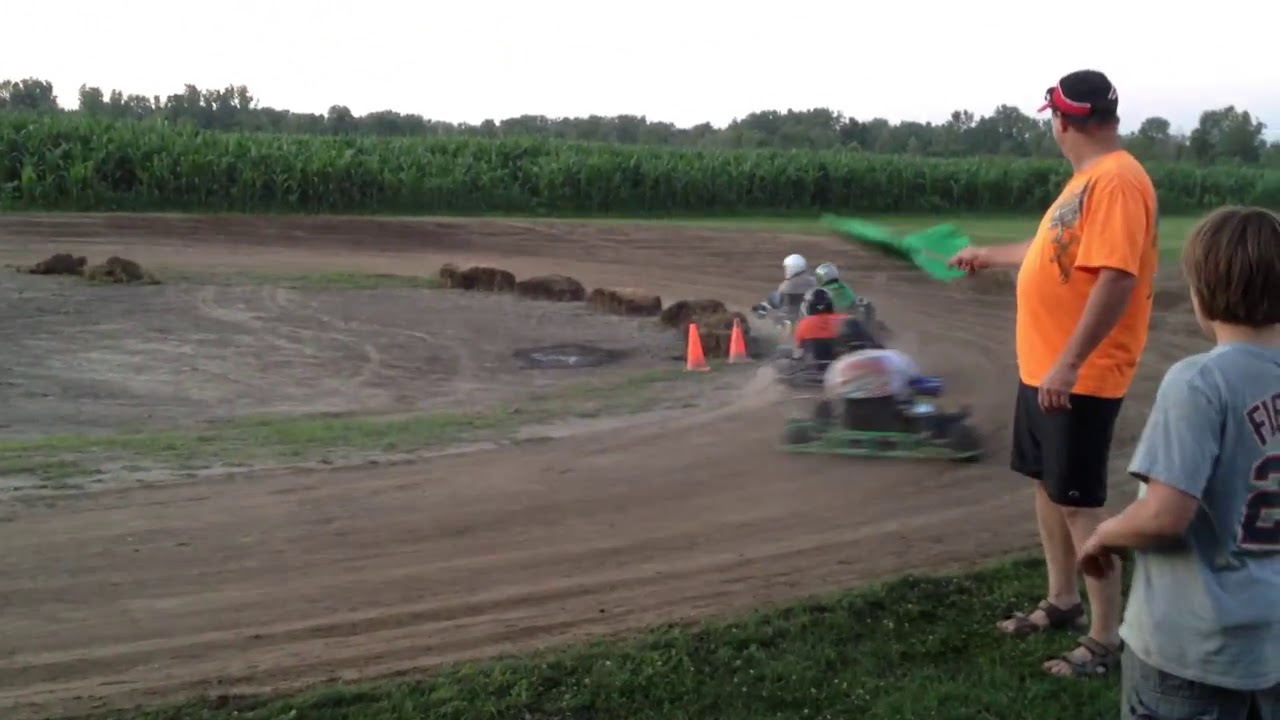The photograph captures a thrilling scene of a go-kart race on an oval-shaped dirt track in what appears to be a farmland, possibly a cornfield, given the organized green plants resembling rows of corn and a distant grove of trees. As the go-karts, four in total, speed around a left turn, the image captures their motion, rendering them somewhat blurry to emphasize their velocity. Cones are strategically placed around the track to prevent crashes. In the foreground, on the right side of the image, a man with a potbelly, wearing an orange t-shirt, black shorts, and a black hat with red on it, watches the race intently. Next to him stands a young boy with medium brown hair, donning a gray t-shirt with partial letters and a number 2 visible on the back, paired with gray shorts. Both spectators are standing on a patch of grass that edges the dirt track, adding a human element to the excitement of the ongoing race.